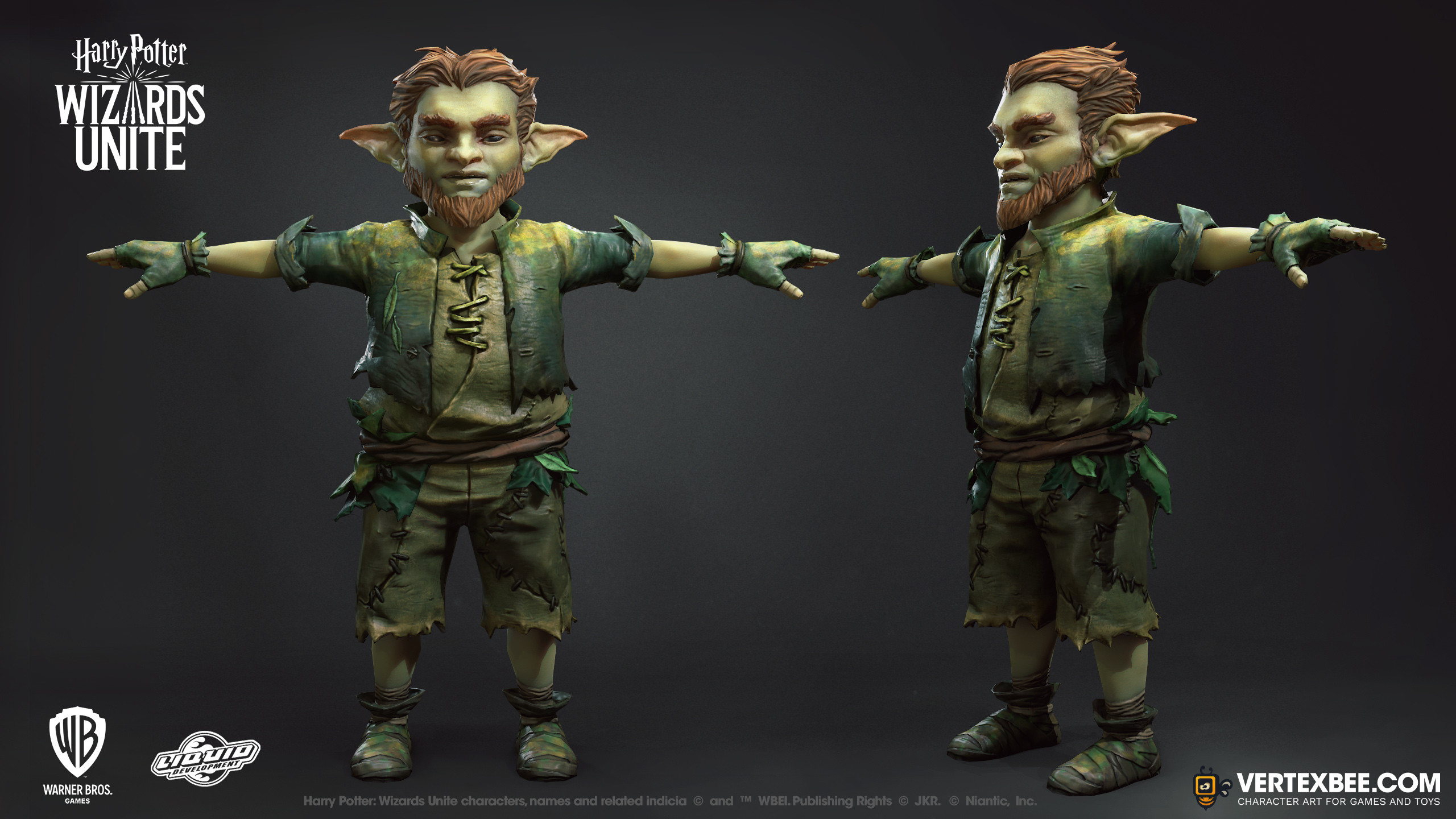A computer-generated character resembling a greenish goblin or hobbit is depicted in intricate detail. With pointy ears jutting out to the sides, the character features slicked-back brown hair and a full brown beard, notable for its lack of a mustache. Dressed in an old peasant outfit, he accessorizes with fingerless gloves and rustic shoes fashioned from sacks, tied around his ankles with ropes. The character is showcased from two different angles, both with arms extended outward. 

In the top left corner, a "Harry Potter: Wizards Unite" logo is prominently displayed. The bottom left corner features the WB (Warner Bros) logo and a Liquid logo adjacent to it. Additionally, a watermark in the bottom right corner reads "vertexbee.com - character art for games and toys."